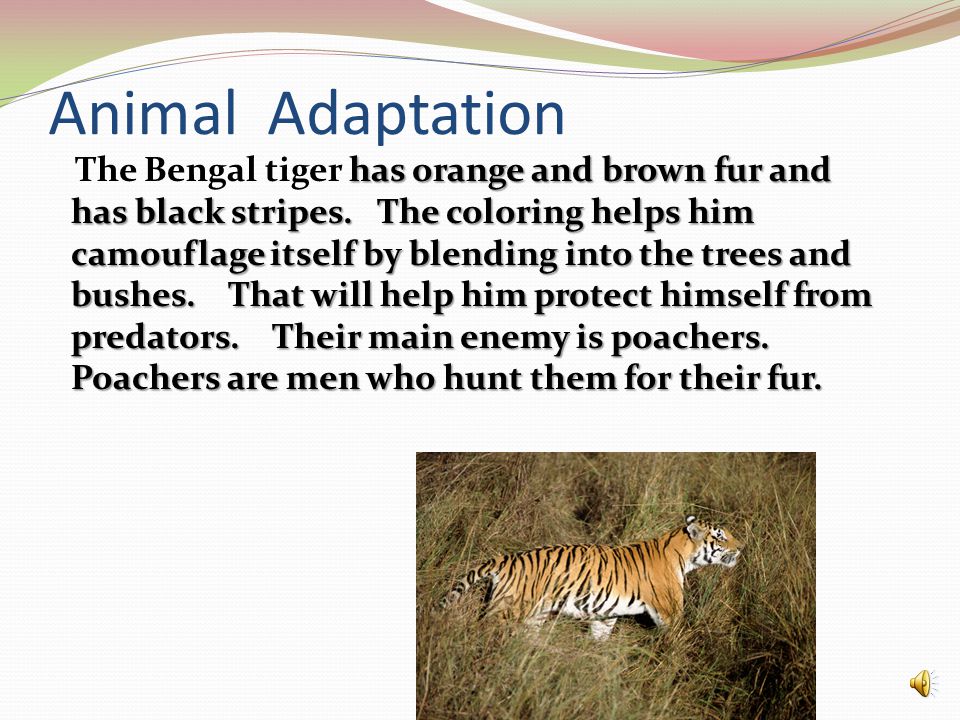The image appears to be a digital slide presentation with a predominantly white background. At the top of the slide is a bold blue title that reads "Animal Adaptation." Just above this title is a decorative flourish featuring swirls of pink, green, and white, adding a touch of visual interest. Directly beneath the title, there is a paragraph in a smaller, solid black font. It describes the Bengal tiger, noting its orange and brown fur with black stripes, which it uses for camouflage among trees and bushes to evade predators. The text also mentions that the tiger's main enemy is poachers, who hunt them for their fur. In the bottom right corner of the slide, there is an image of a Bengal tiger standing amidst dry grass, showcasing its distinctive orange and striped coat with hints of white. Adjacent to the image is a yellow speaker icon, presumably for audio playback of the text. The entire presentation has a minimalistic design, complemented by subtle vertical and horizontal lines on the background, which are faint but discernible.